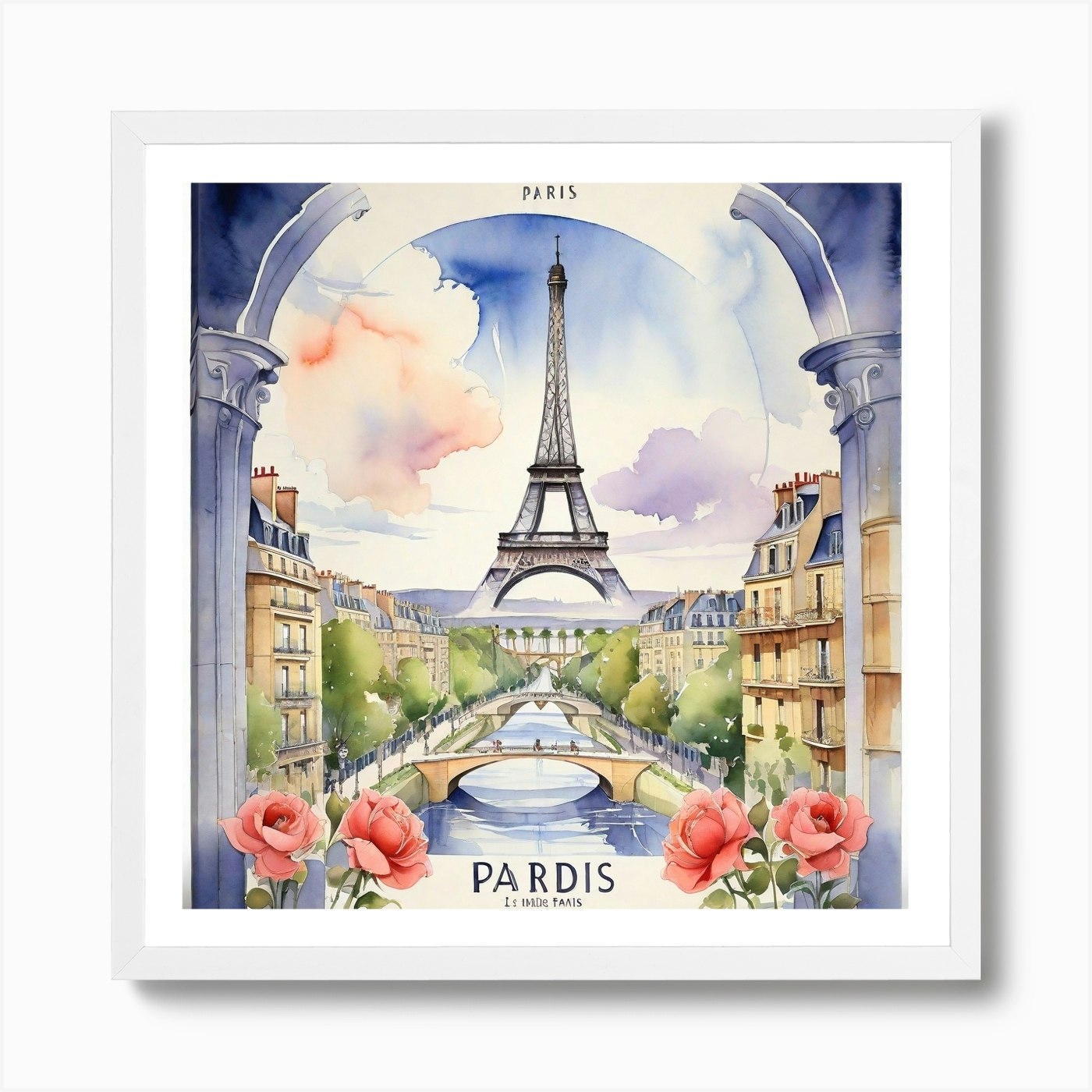The framed poster displayed on a white wall features a detailed watercolor painting of Paris with a light gray border. At the top of the artwork, against a white backdrop, the word "Paris" is prominently displayed in black text. The centerpiece of the painting is a tall, metallic-appearing Eiffel Tower with intricate black etchings. The tower is set against a vibrant blue sky partially covered by a heavy light orange cloud to its left and a purplish one to its right. The scene below is bustling with activity, featuring a mix of three to five-story beige and yellow buildings with blue roofs. Scattered around these structures are lush green trees and various arched stone walkways. A serene waterway flows through the middle of the image, crossed by several tan bridges. In the foreground, the vibrant setting is accentuated by clusters of pink roses on the bottom left and right corners. At the bottom of the painting, the word "P-A-R-D-I-S" is boldly printed in black, framing the entire picturesque Parisian scene.